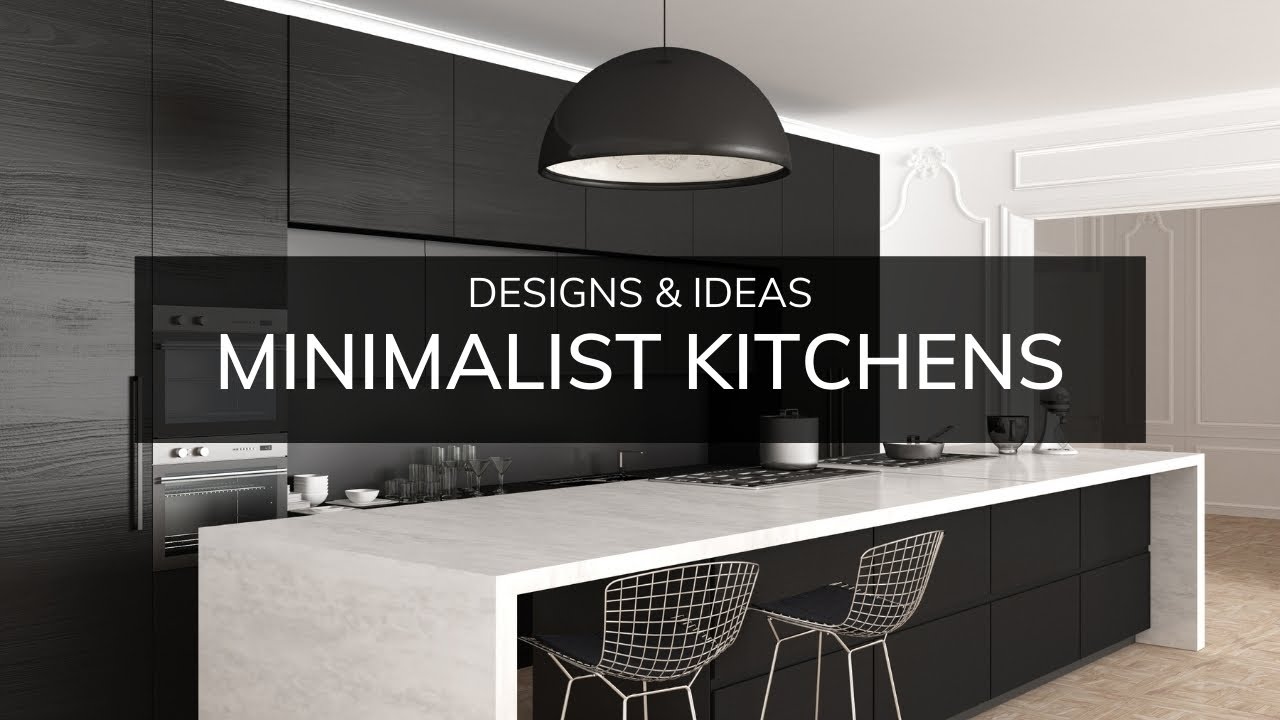The image depicts a modern, minimalist kitchen, predominantly in black and white. Central to the kitchen is a long, white porcelain island with black cabinetry below, which seamlessly integrates the cooking and dining areas. Two metallic chairs are pulled up to the island. Superimposed across the middle of the image, somewhat detracting from the view, are the words "Designs and Ideas, Minimalist Kitchens." The kitchen features sleek, stainless steel appliances, including a built-in double wall oven, and partially visible is a sink faucet. There's a pot on one burner and a pan on another, suggesting the presence of multiple cooktops. Above the island, a black circular hanging light with a white interior provides illumination. The walls remain uncluttered, painted in white, enhancing the minimalist aesthetic. The overall design is very modern, with ample storage provided by drawers under the counter.